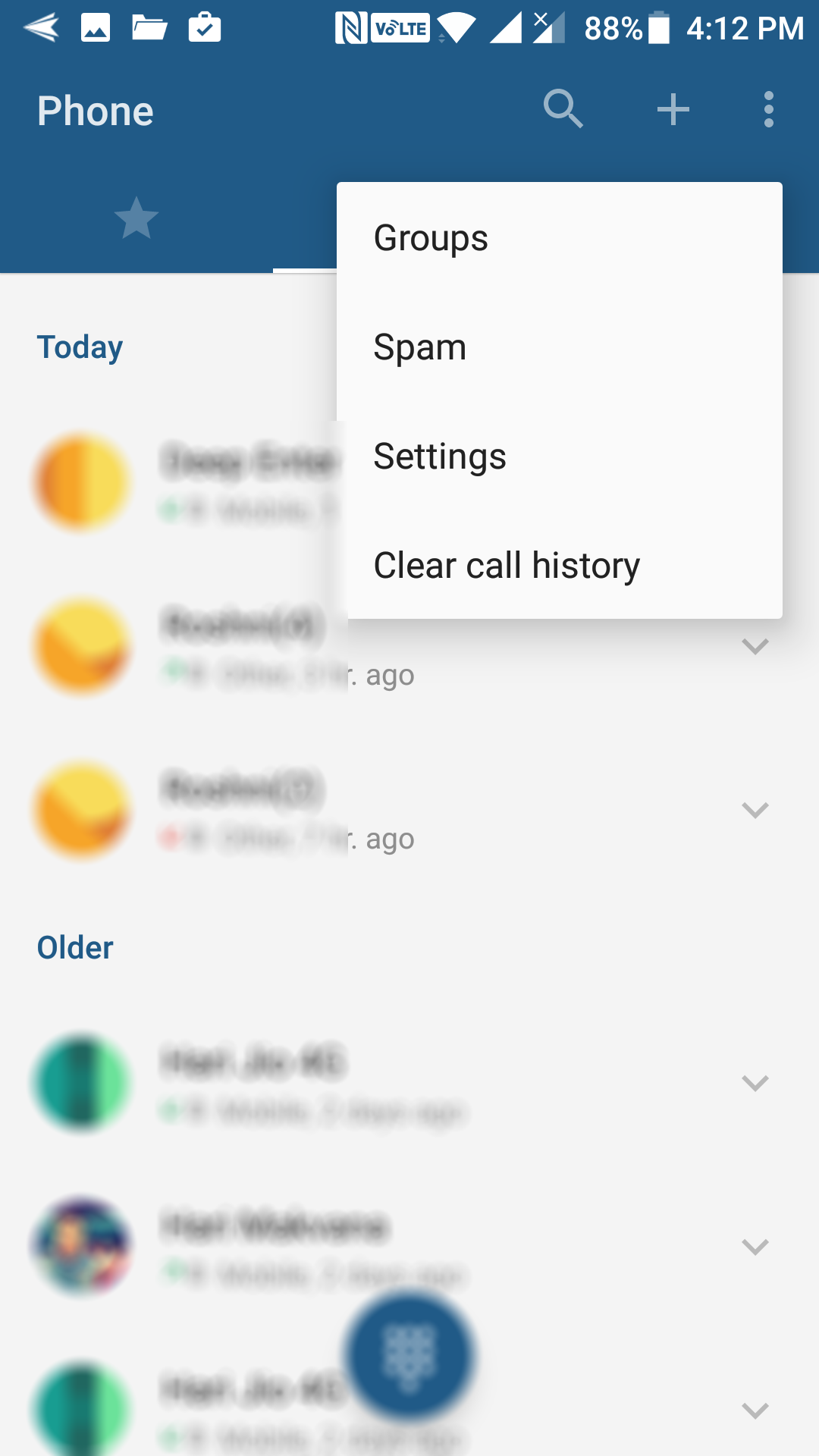In the image, the screenshot depicts a user's phone interface. The top left corner showcases a series of icons including arrows and an image icon, followed by a folder icon featuring a briefcase with a checkmark. Next to these is an unidentified icon labeled "BoLTE", followed by a Wi-Fi signal icon, indicating full connectivity. Adjacent to the Wi-Fi icon are full cellular bars. To the right, the status bar displays "Apple" and a battery meter at 88%, with the time marked at 12:00 PM.

Beneath this blue status bar, there is white text presenting the word "Phone" accompanied by a search icon, a plus symbol, and three vertical dots. Below this, a white box contains options labeled as "Groups", "Spam", "Settings", and "Clear Call History".

Further down, the interface is divided into sections labeled "Today" and "Older". Under "Today", there are three lines each marked with yellow circles beside blurred-out text. Below "Older", two lines are marked with green circles, with the first and third lines indicated, and a blurred-out picture on the second line. Each line in both sections has accompanying black writing next to the icons. At the bottom right, centrally aligned amidst the green circles and the picture, a dark blue button is visible.